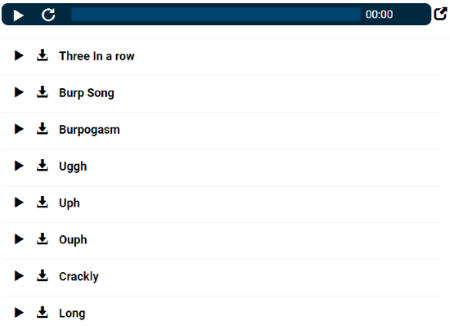The screenshot captures a digital interface, presumably a music or ringtone download platform, displayed against a white background. At the very top, spanning horizontally from left to right, is a dark blue navigation bar. In the leftmost corner of this bar is a white, right-pointing triangle, likely indicating a play button. Just to the right of this triangle is a circular reload icon with an arrow. 

Centrally located within the blue bar, there is a slightly lighter blue text box, hinting at a search or input field. Positioned at the far right of the bar is a timestamp set to "00:00," and adjacent to it is a square icon with an upward-pointing arrow at the 2 o'clock position, possibly for sharing or uploading content.

Below the navigation bar, the interface displays several rows of titles that seemingly represent music clips or ringtones. Each title starts with a black, right-pointing triangle, signaling a play button, followed by a black down arrow with a line beneath it, indicating a download or options menu.

The listed titles, in order from top to bottom, are:
1. Three in a Row
2. Burp Song
3. Burpogasm
4. Ugg
5. Nf
6. Nf
7. Crackly
8. Long